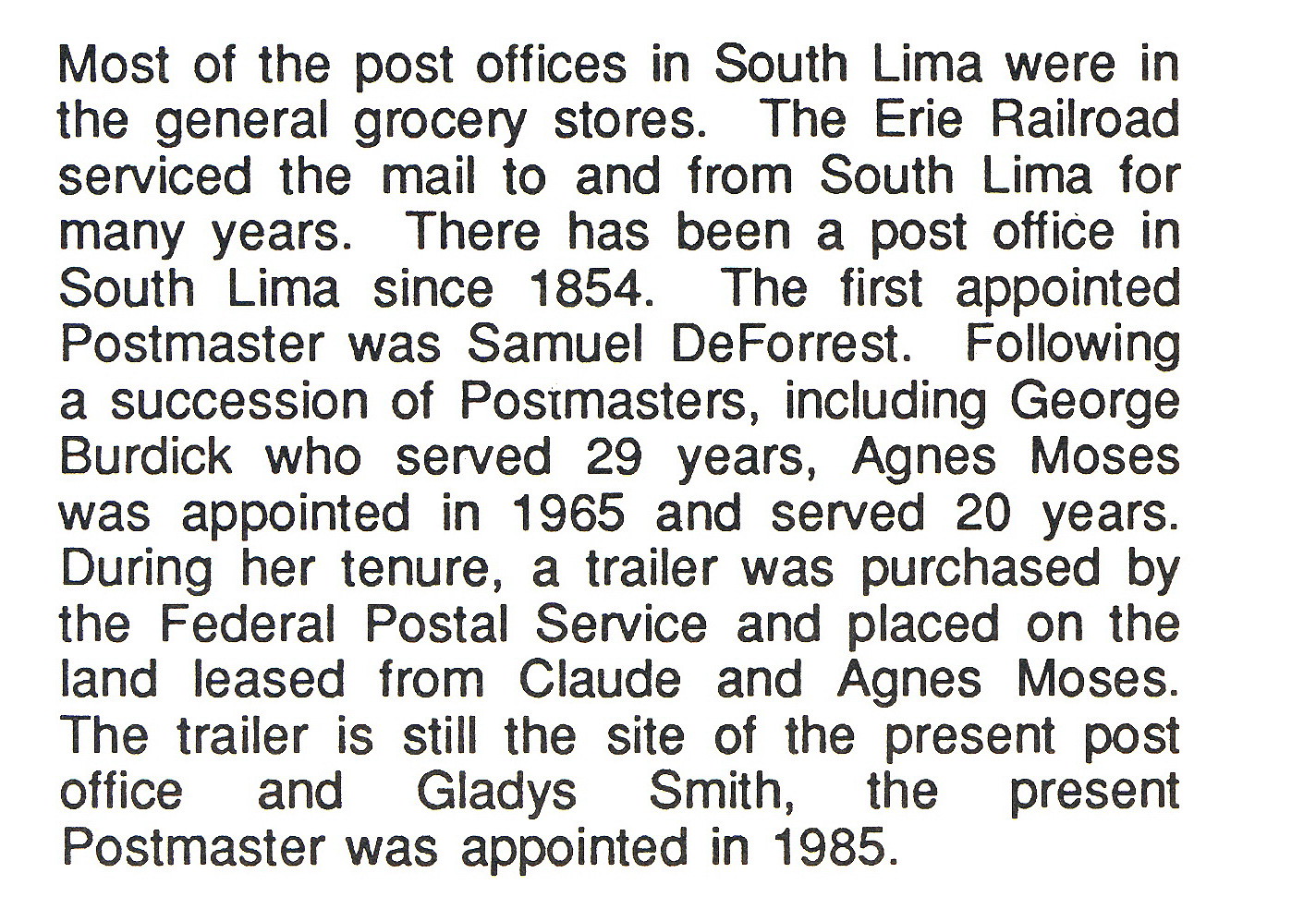The black and white image appears to be a snippet of text from a newspaper or book, taking up the entirety of the image. It details the history of the post office in South Lima. The text explains that most of the post offices in South Lima were located in general grocery stores. The Erie Railroad serviced the mail to and from South Lima for many years. A post office has existed in South Lima since 1854, with Samuel de Forest being the first appointed postmaster. A succession of postmasters followed, including George Burdick, who served for 29 years, and Agnes Moses, appointed in 1965, who served for 20 years. During her tenure, the Federal Postal Service purchased a trailer and placed it on land leased from Claude and Agnes Moses. This trailer still serves as the site of the present post office in Gladys Smith. The current postmaster was appointed in 1985.